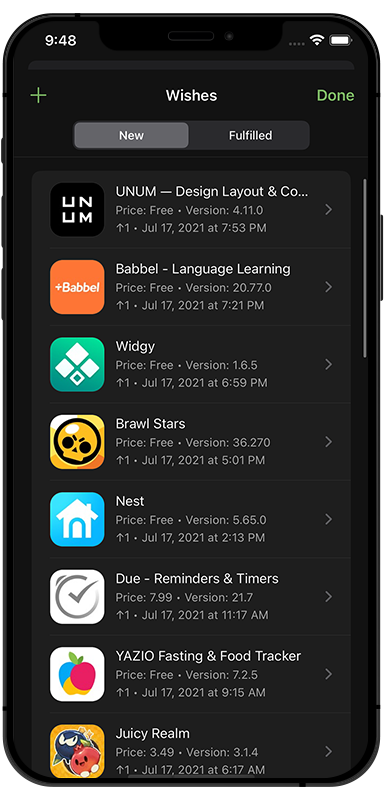The image displays a mock-up of an older iPhone model, showcasing its interface. The iPhone's screen prominently features the time "9:48," alongside full Wi-Fi signal bars and a full battery icon. At the top of the display is a "chin" accommodating the front camera. The main section of the screen shows a labeled interface with the word "Wishes" in white text, flanked by a green plus sign on the left and a green "Done" button on the right.

Beneath the label, two tabs are visible: "New" and "Fulfilled." The "New" tab is highlighted in grey, indicating it is currently selected. This section lists several app icons and descriptions as follows:

1. **UNUM** - A design and layout app, marked as free.
2. **Babbel** - A language learning app with the version number 20.770, listed as free.
3. **Widgie** - An app noted as free.
4. **Brawl Stars** - A free game characterized by a skull logo.
5. **Nest** - Featuring a house icon on a blue background.
6. **Dew** - Represents reminders and timers with a circle and check mark symbol.
7. **Yazio** - Related to fasting and food tracking, indicated by an apple graphic in various colors.
8. **Juicy Realm** - Illustrated with quirky characters wearing crowns, suggesting a game.

This detailed layout and design effectively demonstrate the interface and functionalities of the mentioned apps on this specific iPhone model.